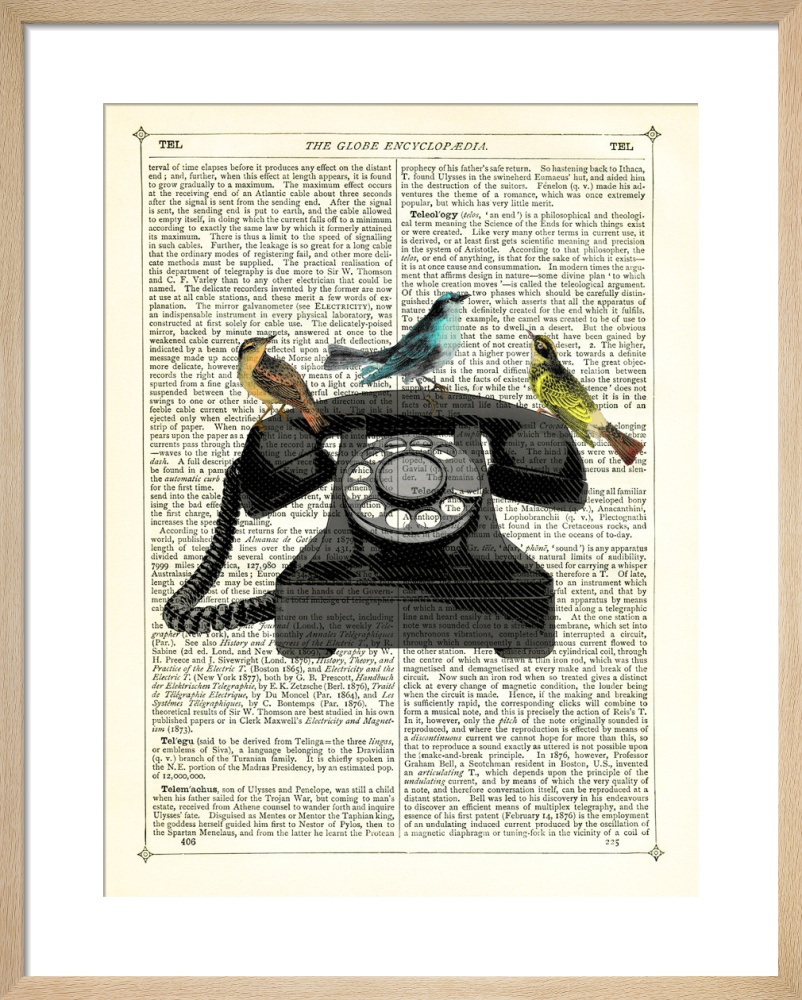This is a photo of a framed encyclopedia page titled "The Globe Encyclopedia." The page is densely packed with long columns of text, including definitions for terms like 'Telugu,' which is said to be derived from 'Telinga.' The page is bordered by decorative four-pointed stars in each corner. Superimposed on the text in the middle of the page is the image of a semi-transparent black rotary telephone, upon which sit three colorful birds: a yellow-orange bird, a blue-teal bird, and a neon-yellow bird. The overall effect gives the impression of a vintage infographic, blending textual knowledge with artistic overlay.